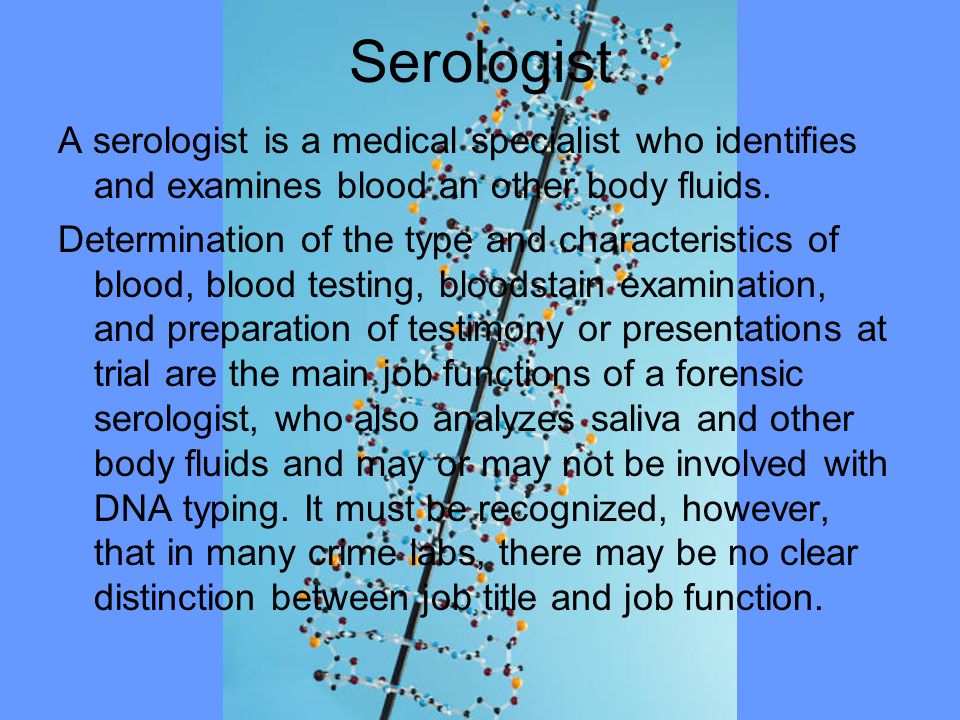The image is an informational slide with a background featuring two purplish-blue rectangles on the left and right sides, and a light blue rectangle in the center that is slightly larger than the side sections. In the middle section, various colored dots (yellow, red, green, and blue) are connected by white lines, resembling a DNA strand. Overlaid on this central image is black text. The large text at the top reads "Serologist," followed by detailed smaller text that describes the role: "A serologist is a medical specialist who identifies and examines blood and other body fluids. Determination of the type and characteristics of blood, blood testing, blood stain examination, and preparation of testimony or presentations at trial are the main job functions of a forensic serologist, who also analyzes saliva and other body fluids and may or may not be involved with DNA typing. It must be recognized, however, that in many crime labs there may be no clear distinction between job title and job function."